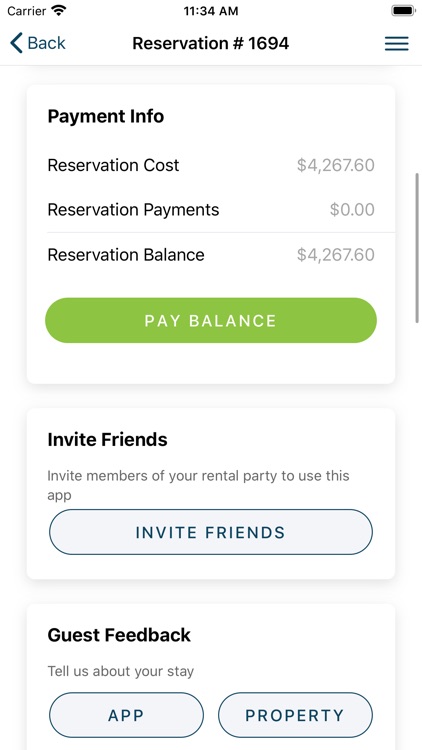Screenshot of a smartphone screen displaying a detailed reservation and payment interface. The screen is a tall rectangle with a status bar at the top. On the left side of the status bar, it displays the word "carrier." On the right side, there's a battery icon, and in the center, the time is shown as 11:34 a.m. Beneath the status bar, the heading reads "Reservation #1694" with a "Back" arrow on the left and a menu icon with three stacked lines on the right.

Below the heading, a white square contrasts against the black background. The title "Payment Info" stands prominently at the top of this section, followed by three lighter subheadings: "Reservation Cost," "Reservation Payments," and "Reservation Balance." Adjacent to the subheadings are the respective amounts: $4,267.60, $0, and $4,267.60. 

A prominent long green button labeled "Pay Balance" encourages action beneath these details.

Further down the screen, another white square contains an "Invite Friends" section. Below this, in smaller text, it instructs, "Invite members of your rental party to use this app." A long gray button labeled "Invite Friends" allows users to send invitations.

Continuing down, a white button titled "Guest Feedback" prompts users to provide feedback about their stay. Below this, a prompt "Tell us about your stay" invites more detailed comments.

At the bottom, there are two long arrow buttons labeled "App" and "Property," likely linking to additional information or actions related to the application and the rented property respectively.